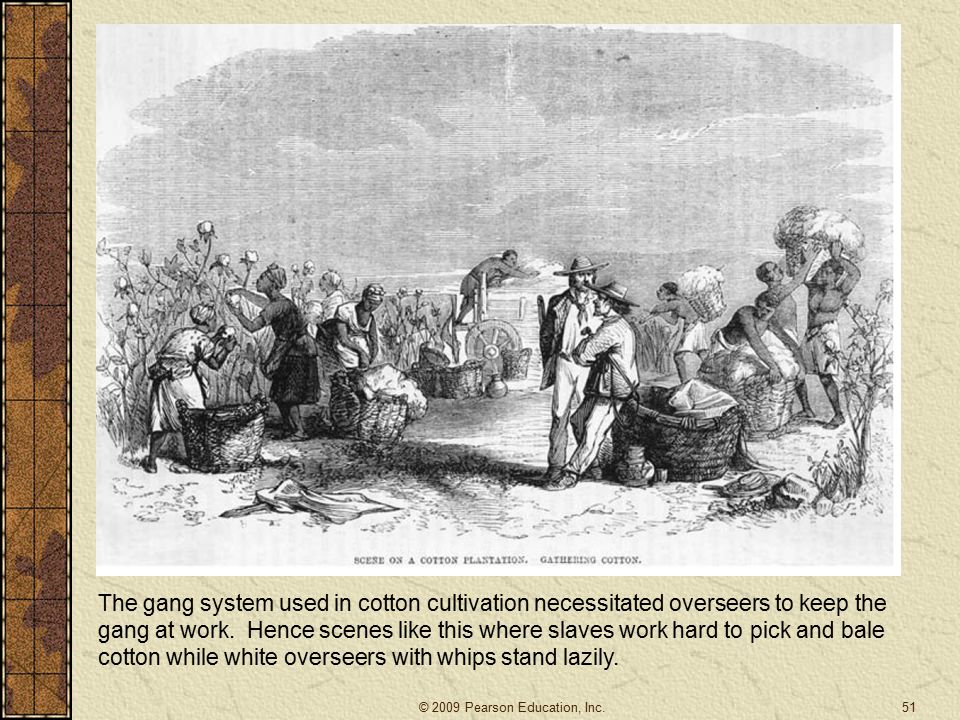The black and white drawing depicts a scene of intense labor on a cotton plantation, highlighting the entrenched system of forced labor. On the left, a group of African-American women, identifiable by their headscarves, diligently harvests cotton and places it into large baskets. In the foreground, two white men dominate the scene: one is standing, dressed in a hat, tie, and suit, and appears to be in conversation with the other, who is similarly dressed and sitting on the edge of a large basket. The middle ground reveals a man loading goods onto a vehicle, with the wheel of the vehicle partially visible. On the right side of the image, four robust African-American men are seen hoisting heavy baskets, preparing to load the cotton onto the vehicle. Beneath the image, text explains the "gang system" used in cotton cultivation, which required overseers to supervise and ensure continuous labor. The caption underscores the stark contrast between the hard-working slaves and the white overseers who stand idly by, often resorting to whips to enforce labor.